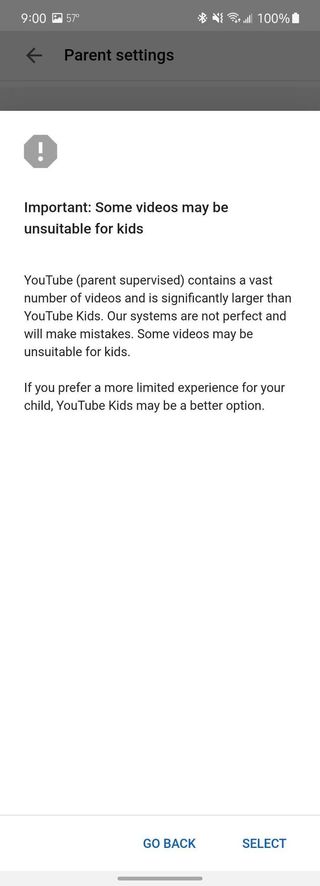This image is a screenshot of a "Parent's Settings" page within an application. Overlaying the settings page is a prominent pop-up alert box. 

The alert is visually critical, marked by a grey octagon with a central exclamation point icon in the top left, signifying caution. Under this icon, there is a bold black font message warning, "Some videos may be unsuitable for kids. YouTube parent supervised contains a vast number of videos and is significantly larger than YouTube Kids. Our systems are not perfect, and we will make mistakes. Some videos may be unsuitable for kids. If you prefer a more limited experience for your child, YouTube Kids may be a better option."

At the bottom of the pop-up, on the lower-right side of the screen, two interactive options are visible: "Go back," which is underlined and written in blue, and to its right, "Select," which is also in blue. There is also a small grey bar underneath the "Go back" button suggesting it as a default or primary action.

In the background, partially visible through the semi-transparent alert box, the settings page header reads "Parent Settings" in black with a left-pointing arrow next to it, indicating a navigational option to return to the previous menu.